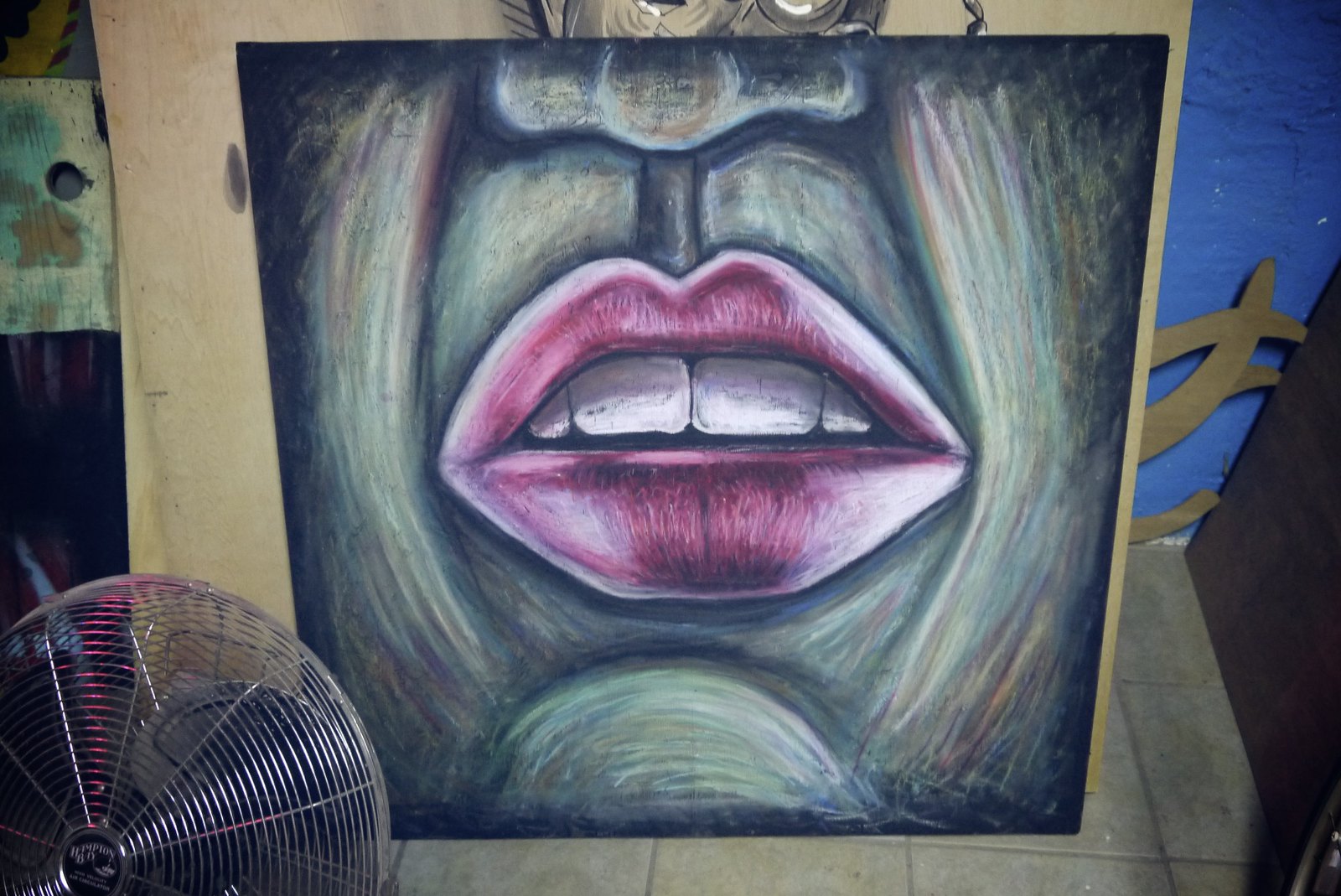A close-up image captures the blurred face of an individual standing against an outdoor wall. The person has noticeable pink lips and a partial view of their white teeth, specifically the front two and the ones adjacent to them. In the bottom left corner, a silver-bladed fan is visible, adding an industrial touch to the scene. The stone-tiled floor beneath shows an array of scratch marks and paint splatters in various colors including white, black, gray, and red. In the bottom right corner, there are curved objects whose shapes add an intriguing element to the composition. The background on the right side of the image hints at an outdoor environment.